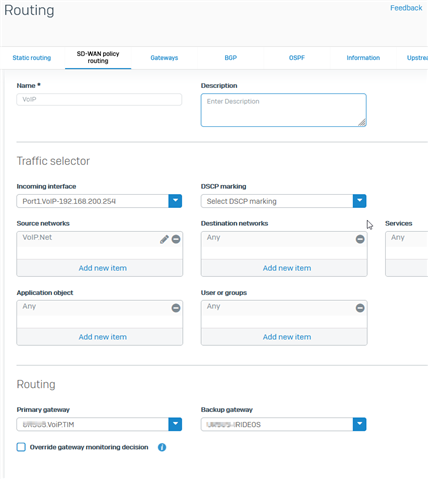Screenshot of a website page displaying routing options

In this detailed screenshot of a website interface, the topmost section is a gray box containing two headers. On the left side of the box, bold, black text reads "Routing," while the right side features "Feedback" in smaller, blue text. Below this, a narrow white line spans the width of the page, separating the header from the main content area.

The main content consists of multiple menu options or buttons aligned horizontally. From left to right, these options include Static Routing, SD-WAN Policy Routing, Gateways, BGP, OSPF, and Upstream, though some titles are partially cut off. Notably, the SD-WAN Policy Routing button stands out in black with an underline, indicating it is the selected option, while the other buttons are in blue.

Continuing down the page, the layout alternates between gray boxes and white spaces. The first section is labeled for entering a "Name" and "Description." Following this is a section titled "Traffic Selector," containing several boxes with different configuration options. Further down, another section called "Routing" appears, offering fields for designating a "Primary Gateway" and a "Backup Gateway." The screenshot cuts off at this point, providing a partial, yet detailed view of the routing configuration interface.